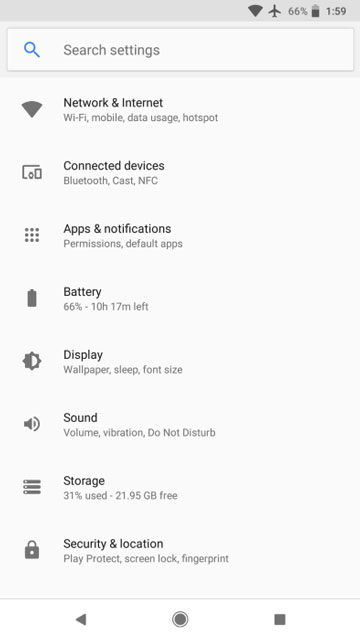This is a detailed screenshot of a mobile device's settings menu. At the very top of the image, there is a gray status bar displaying the current Wi-Fi signal strength, an airplane mode icon, a battery life indicator at 66%, and the time, which is 1:59 PM. Below the status bar, a search bar is visible with a blue magnifying glass icon and the placeholder text "Search settings."

The settings menu is organized into several sections. The first section, "Network & internet," includes options for managing Wi-Fi, mobile data, data usage, and hotspots, all represented by a Wi-Fi symbol. The next section, "Connected devices," includes options for Bluetooth, casting, and NFC (Near Field Communication).

Following this, there is a section for "Apps & notifications," which covers app permissions and default apps, visually indicated by a grid of nine circles. The "Battery" section shows that the device has 66% battery life remaining with an estimated 10 hours and 17 minutes left, accompanied by a battery icon.

Further down, the "Display" section offers settings for wallpaper, sleep mode, and font size, marked by a sun icon with a black center. The "Sound" section features options for volume, vibration, and Do Not Disturb mode, represented by a speaker icon. 

Lastly, the "Storage" section indicates that 31% of the device's storage is used, leaving 21.95 GB free, and features a lock icon labeled "Security & location."